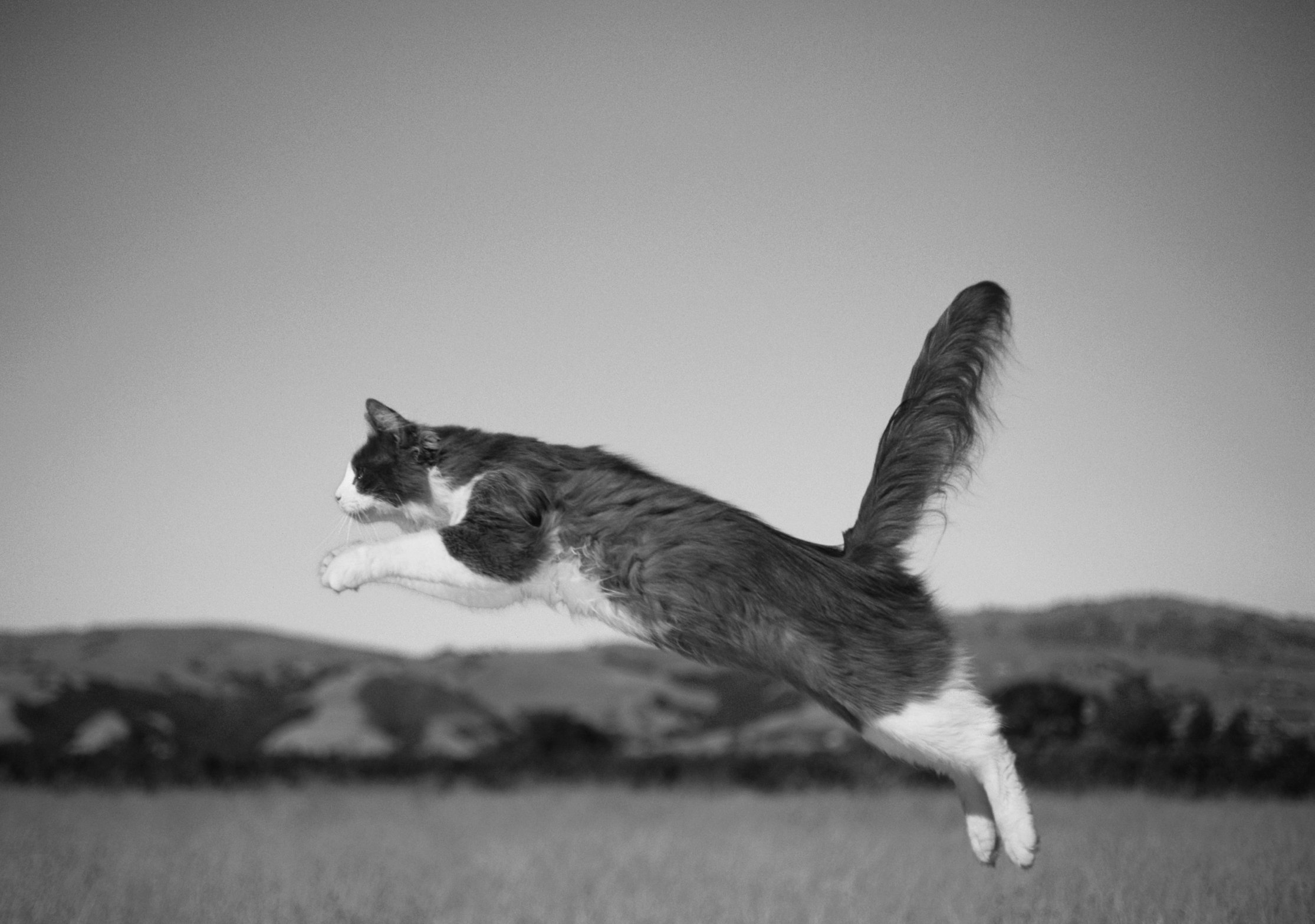This black-and-white photograph captures a striking moment of a cat in mid-leap, creating the illusion of flight. The cat, appearing to be a multi-colored feline likely with patches of gray, white, or black, is fully stretched out in profile from right to left. Its front paws extend forward and its back paws trail behind, while its tail stands straight up, perpendicular to its body. The cat's ears are alert and pointed up, indicative of its focus. The background shows a blurry landscape consisting of grassy hills and a gray sky, emphasizing the cat's dynamic motion. The photo's central focus remains on the cat, illustrating its fluid movement and the grace of its leaping posture.